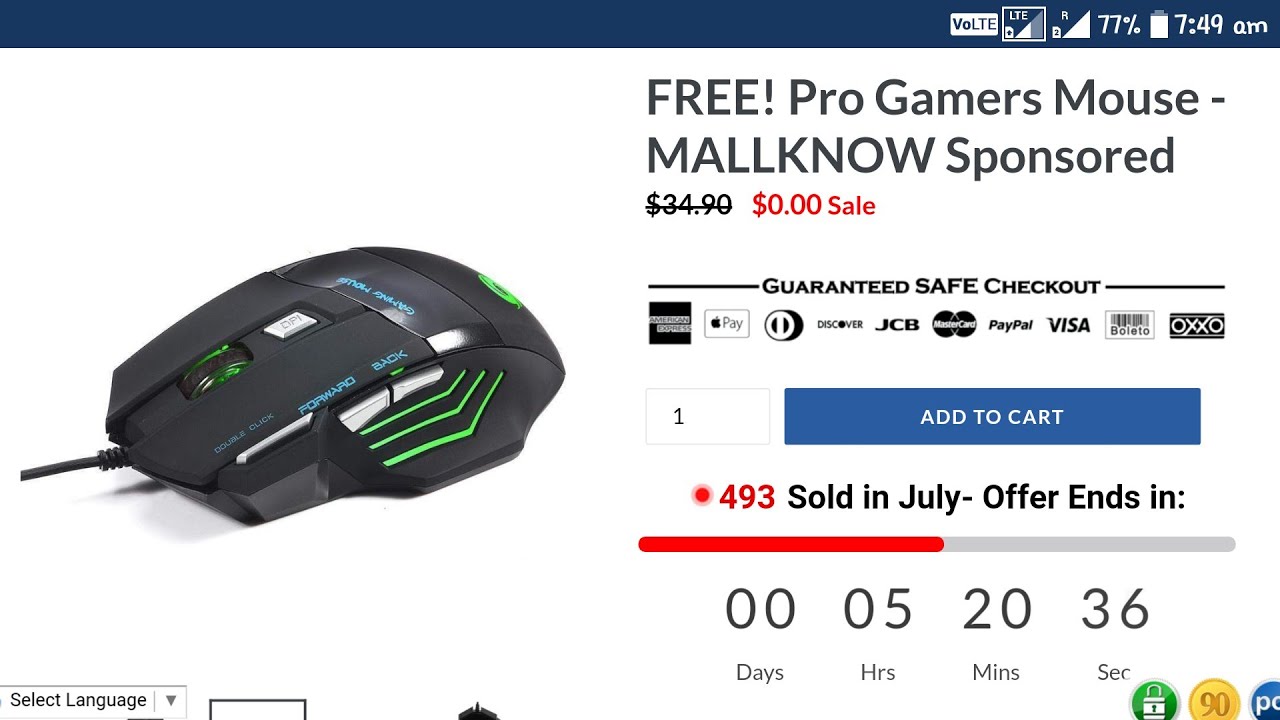The image displays a cell phone or tablet screen with an advertisement for a gaming mouse. The top of the screen features a dark blue band. On the right side of this band, white icons indicate the cell phone's connection status, battery level at 77%, and the time, 7:49 AM, along with "VOLTE" and a rectangle with "LTE" and half a triangle inside.

The page background is predominantly white. Towards the top right, black uppercase letters spell out "FREE!" followed by "Pro Gamers Mouse" in regular lettering. Below this, "MALLKNOW" is written in uppercase letters with "sponsored" right under it. 

The next line shows a price of $34.90, crossed out, with "$0.00 sale" highlighted in red next to it. Below that, the text "Guaranteed Safe Checkout" is accompanied by icons for American Express, Apple Pay, Discover, JCB, MasterCard, PayPal, Visa, Boleto, and OXXO, all in dark ink.

Further down, there is an open rectangle with the number "1" inside. To its right is a blue rectangle with white lettering that reads "Add to Cart." Below that, red text lists $4.93, followed by black text reading "Sold in July, Offer Ends In." A progress bar below this is half red and half gray. Under the progress bar, a countdown timer details "00 days, 05 hours, 20 minutes, 36 seconds." The image cuts off at the bottom of the screen after this point.